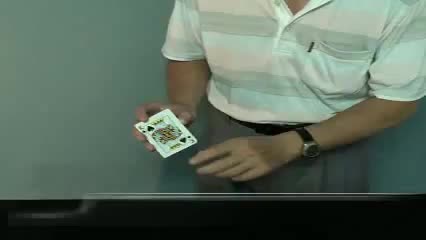In the photograph, a man is prominently displaying a King of Spades poker playing card towards the camera with his right hand. He is dressed in a stylish, light-colored polo shirt featuring horizontal stripes of pink, gray, and blue. The shirt has a turndown collar and short sleeves, with the top three buttons open, revealing a bit of his chest. A small chest pocket, detail further enhances the shirt's casual look. On his left wrist, the man sports a sleek watch with a black band, a black watch face, and a silver rim.

The backdrop consists of a very slightly greenish-gray wall, which adds a neutral tone to the image. At the bottom, there's a black border, possibly a photographic glitch. The photograph focuses only on the man's torso, cutting off his face and shoulders. The King of Spades card he is holding has a stylized cartoon image of a king and the spade symbols strategically placed in the top right and bottom left corners. The overall composition centers on the visual impact of the card and the man's casually stylish appearance against the simple background.